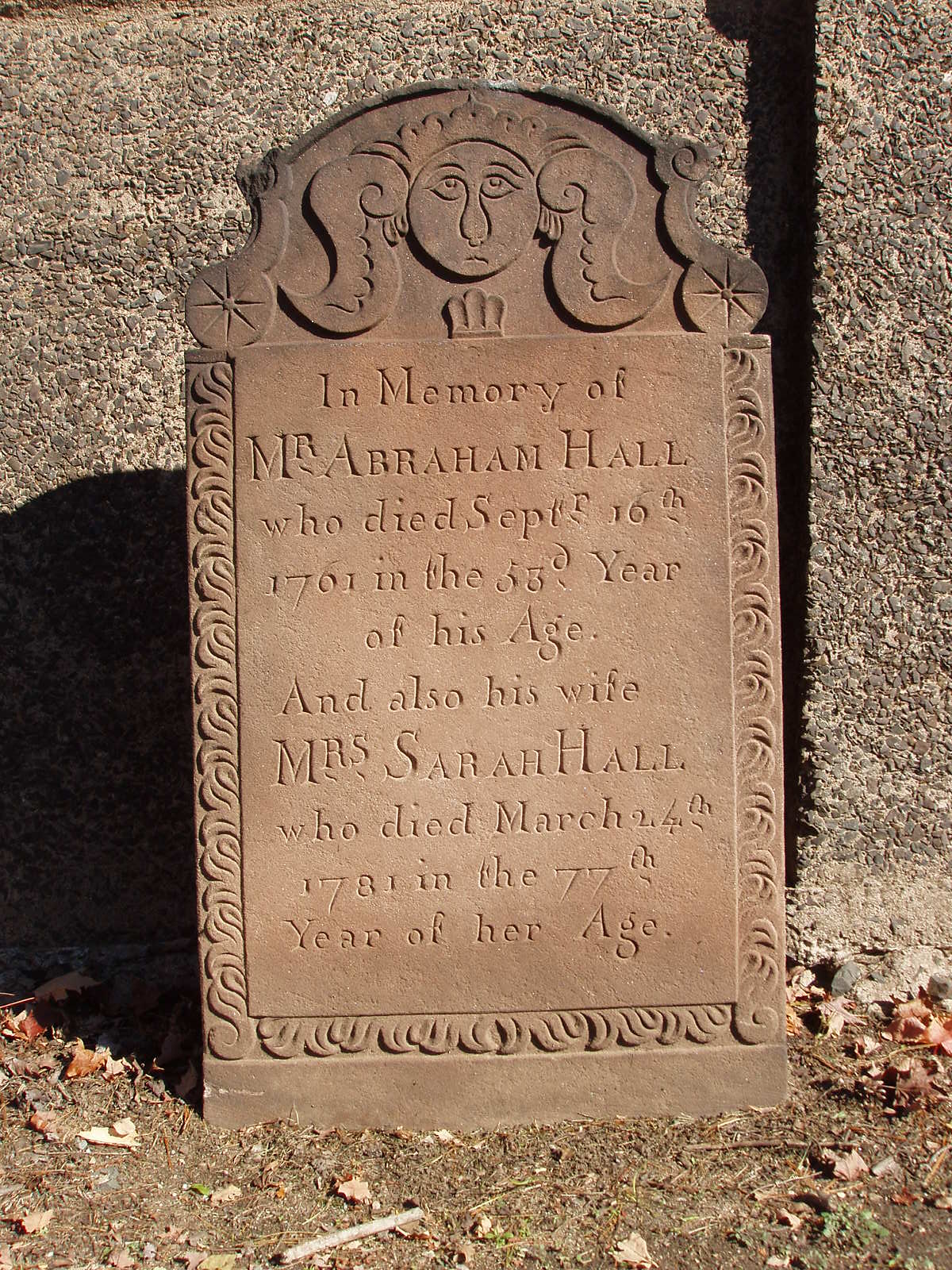The image features an aged gravestone, maroon in color with a darker hue at the top. The gravestone commemorates Mr. Abraham Hall, who died on September 16, 1761, in the 53rd year of his life, and his wife, Mrs. Sarah Hall, who passed away on March 24, 1781, at the age of 77. At the top of the headstone is a carved depiction of a face with a sad expression, flanked by what appear to be either horns or stylized hair. There are also wing motifs and elaborate design elements around the sides and bottom of the marker. The gravestone stands against a backdrop of a stone wall. The ground in front of it is primarily composed of dirt, dry leaves, and some sparse, brown grass, suggesting a dry environment possibly in the fall season.